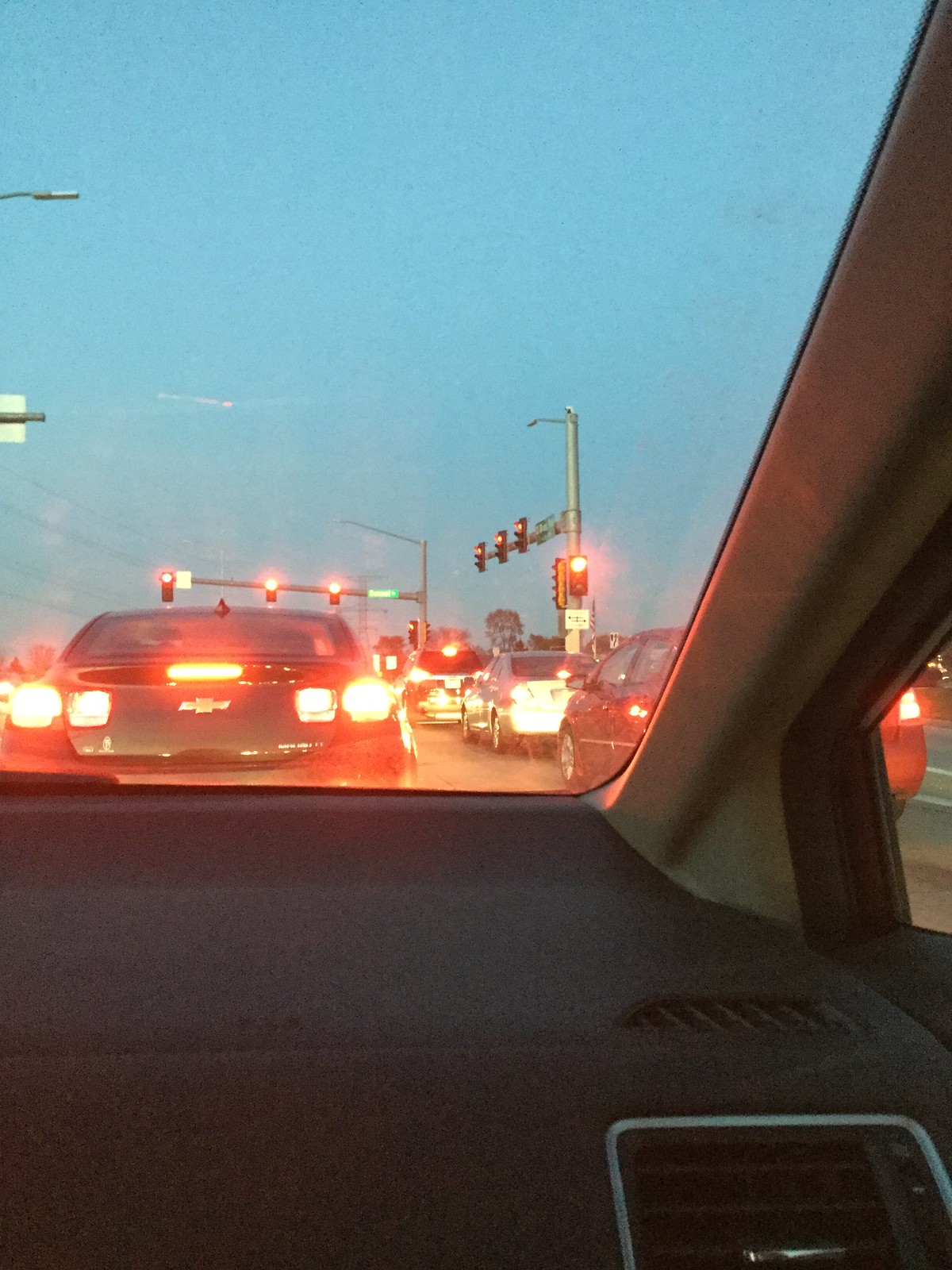The photo, taken from the passenger side of a vehicle through the windshield, vividly captures a moment at a red light during dusk. The sky is blue, suggesting the sun has just set or is about to. Streetlights, although present, remain unlit. The image features six cars in total, all illuminated by the red glow of multiple traffic lights. Directly in front is a black Chevrolet Malibu sedan. To its right is a red sedan, followed by a silver sedan, and then a black CUV up ahead. The vehicle's interior features a black dashboard and a beige or gray A-frame. Trees can be seen in the distance, adding context to the urban setting. A street sign is also visible near the traffic lights at the cross street, all emitting a red signal, indicating a complete stop for all directions of traffic.